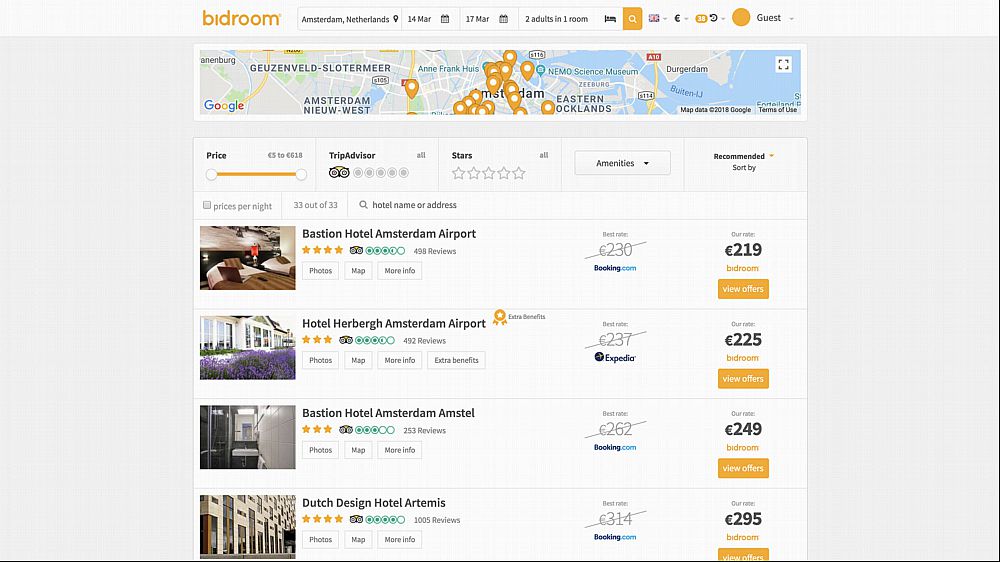The image depicts a booking application called "Bedroom," where a user is searching for accommodations in Amsterdam, Netherlands. The search parameters are set for a stay from March 14th to March 27th for two adults in one room. At the top of the screen, there are various search options, including a detailed map of the Amsterdam area highlighting potential lodging alternatives. This map, integrated with Google Maps, allows users to zoom in and out for better navigation. Below the map, a series of small images display different hotel options, each accompanied by pricing information. These hotels are sorted from the most affordable to increasingly expensive. Users can adjust the visible price range using a draggable gauge to filter results based on their budget. Additionally, there are options to filter hotels by TripAdvisor reviews, although it appears this search did not incorporate review criteria.